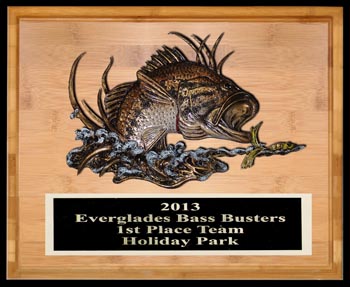This image depicts a detailed and ornate wooden plaque celebrating a fishing achievement. The plaque features a prominent illustration of a large fish, characterized by its brown and silver hues, and covered with numerous spines or barbels on its head. The fish is shown dramatically leaping out of bluish-silver water, its mouth wide open as it attempts to catch a yellowish-green lure. This action is set against a dual-toned wooden backdrop, with a lighter brown central area and a darker brown border. Below the vivid depiction, a black rectangle with white text prominently displays the award inscription: "2013 Everglades Bass Busters First Place Team Holiday Park." The intricate combination of elements provides a dynamic and vivid visual narrative, embodying the excitement of the fishing triumph celebrated by the plaque.